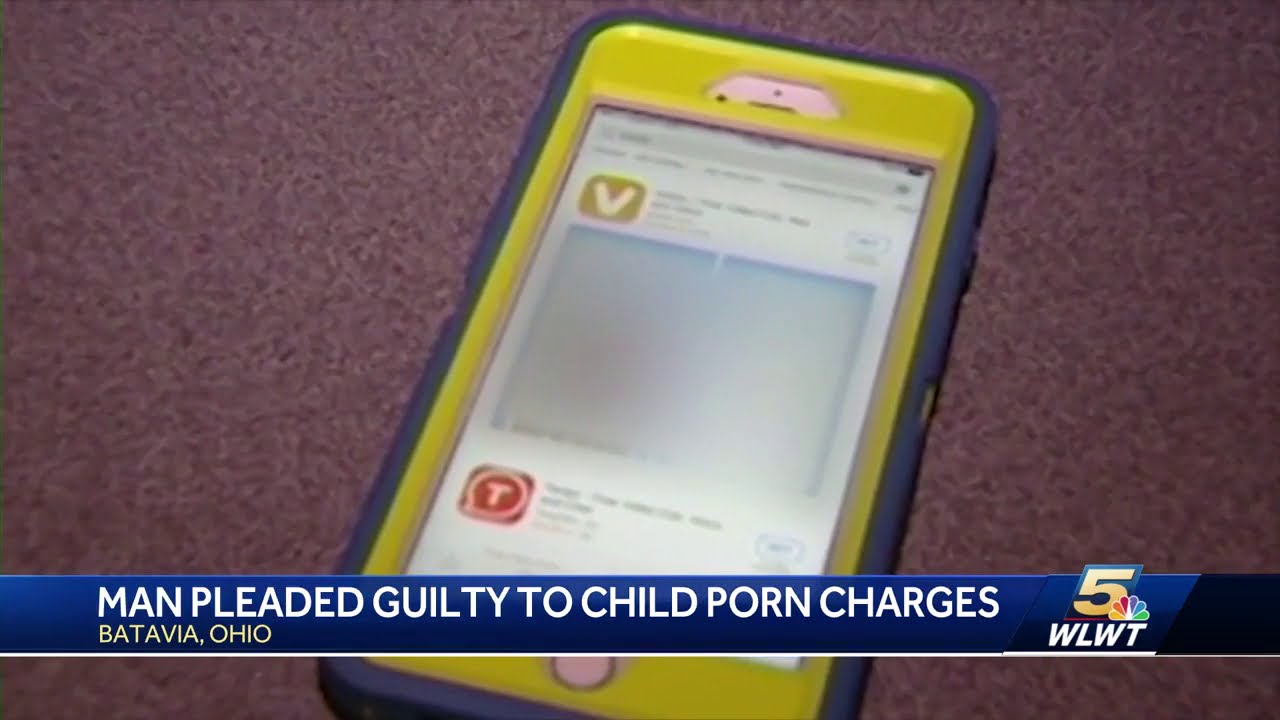This image is a still frame taken from a local news broadcast on WLWT, an NBC-affiliated station. It features a blurred-out smartphone displaying social media posts, encased in a distinctive yellow hard shell with gray edges, sitting on a pinkish-grayish Formica countertop. A blue banner runs along the bottom of the screen with the headline in white text: "Man Pleaded Guilty to Child Porn Charges," and just below it, "Batavia, Ohio" in yellow text. On the right side of the banner, the channel's emblematic golden "5" is shown, accompanied by the NBC Peacock logo. The phone screen itself appears to show a mustard-yellow square with a "V" on it and a red square with a "T," though the details are blurred.